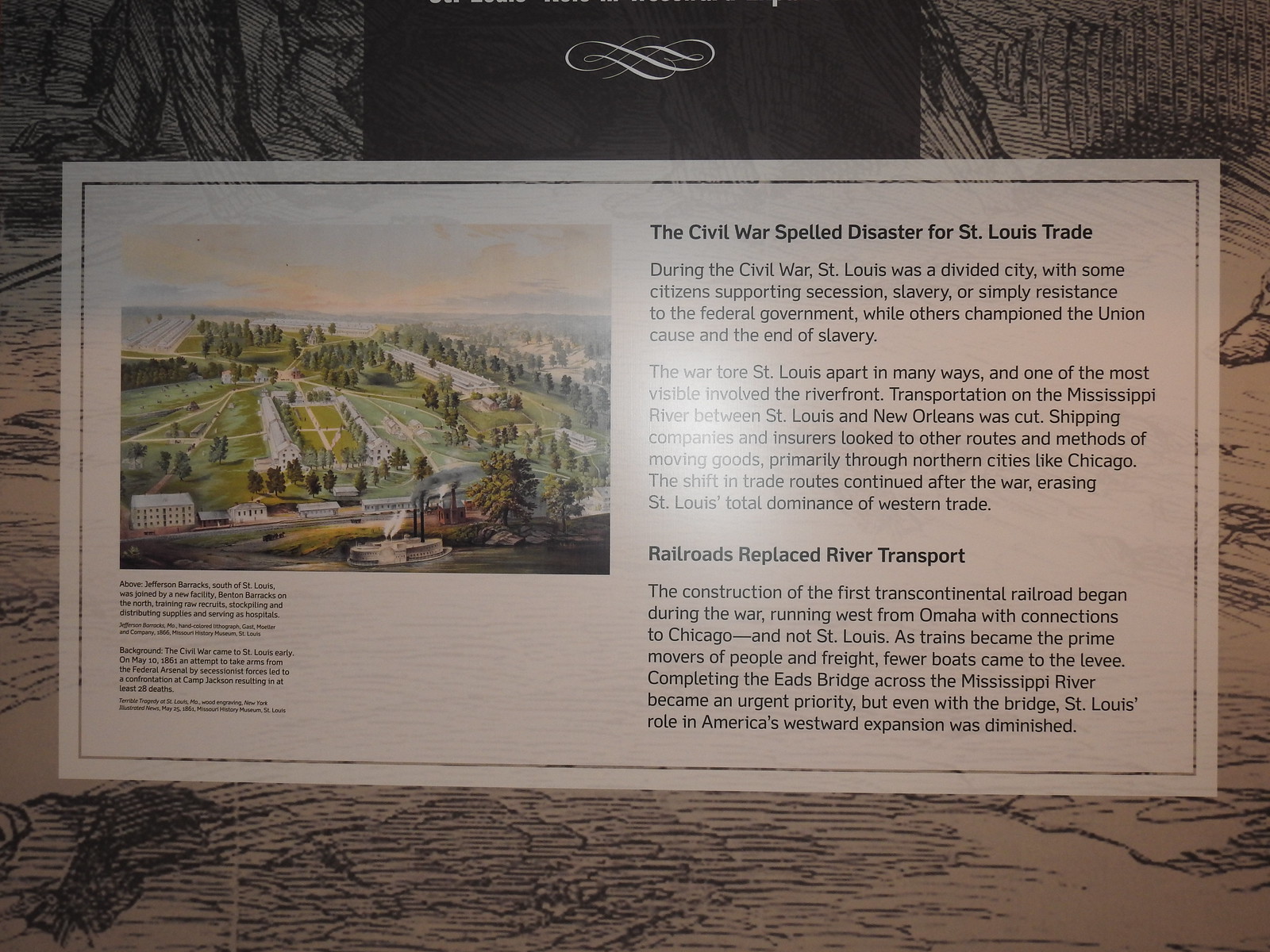The image is an indoor photograph of a horizontally oriented informational placard, designed with a photographic representational realism style. The placard has a light gray background and is divided into two vertical columns. The left column features a detailed color illustration of an overhead view of St. Louis, situated on the banks of the Mississippi River, with a prominent paddle boat steamship on the water. Below this illustration, two pieces of aligned text provide further context.

The right column contains two main sections of text, each highlighted with bold headings. The first section, titled "The Civil War Spelled Disaster for St. Louis Trade," describes how the Civil War caused a significant divide in St. Louis, affecting its riverfront and trade routes. The text explains how the conflict disrupted transportation on the Mississippi River between St. Louis and New Orleans, leading shipping companies to seek alternative routes, primarily northward to cities like Chicago. This shift continued post-war, diminishing St. Louis's dominance in western trade. The second section, "Railroads Replaced River Transport," details how railroads eventually overtook river transport in prominence. It mentions the urgency to complete the Eads Bridge and how trains became crucial for moving freight and people, further diminishing St. Louis's role in America's westward expansion.

The background of the placard features a beige wood grain texture with black hatch marks and a central white scroll design at the top, adding a historical and elegant touch. The informative text is carefully crafted to provide a comprehensive understanding of St. Louis's trade transformation during and after the Civil War, highlighting significant events and changes in transport logistics.